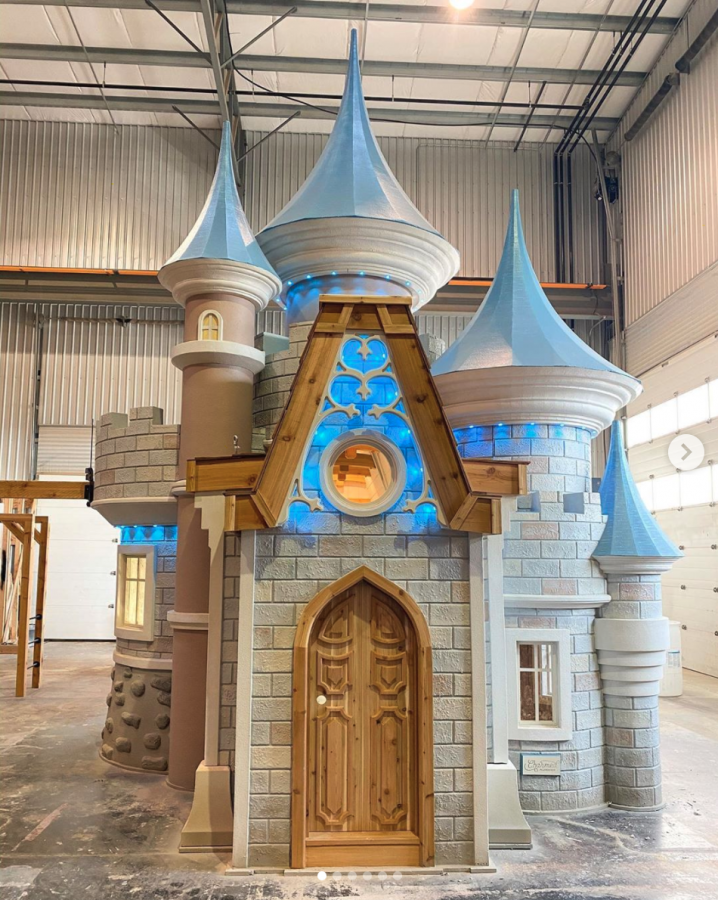The image depicts a whimsical, Disney-inspired playhouse castle, set in a spacious factory or large garage-like environment with makeshift walls. The structure is predominantly gray, resembling granite bricks, with vibrant blue tower roofs, and features elements of sandy brown, orange, neon blue, and gray tones. The wooden door, adorned with intricate carvings, sits beneath a large arch, and above it are stained glass windows. The castle includes several towers and steeples with balconies, enhancing its playful and magical appearance.